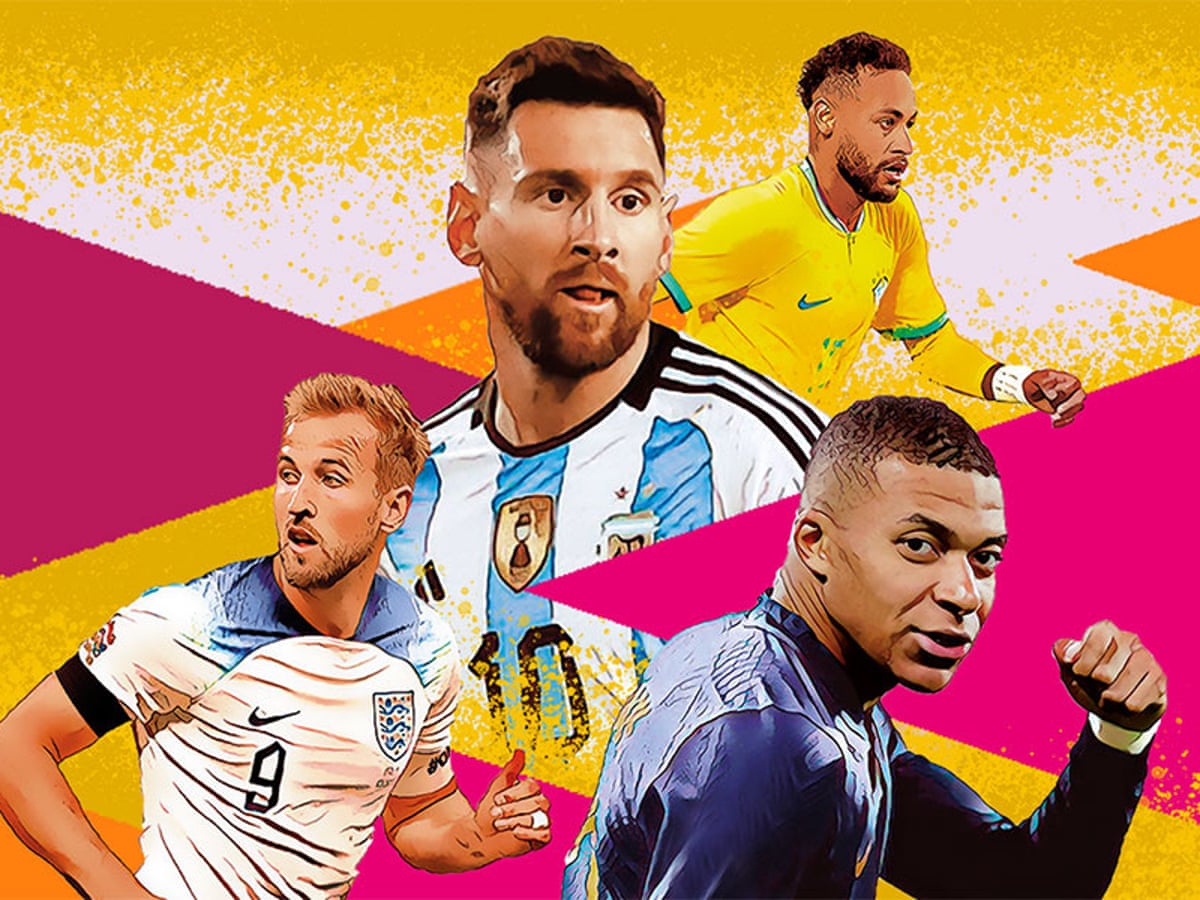The image is a vibrant, borderless square collage featuring four distinct soccer players rendered in a stylized, cartoon or hand-drawn effect, giving the impression of a mix between digital painting and photograph. The background is predominantly yellow adorned with orange-pink triangles all around. At the top, an African male player is depicted in a yellow jersey with green stripes on the sleeves, looking to the right. Beneath him, the central figure is a Caucasian male with reddish-brown hair, dressed in a white and blue striped jersey prominently displaying the number 10. The bottom left corner showcases another Caucasian player in a short-sleeved jersey featuring blue shoulders and a large black 9 on the front, complemented by a Nike swoosh and a coat of arms. The final player in the bottom right is an African male in a long-sleeved blue jersey with subtle white patterns and yellow accents, his left arm bent and fist slightly raised. The collage's intricate background, with fading yellow paint splotches and strategically placed colorful triangles, enhances the dynamic and spirited essence of the soccer players, suggesting the artwork could be inspired by modern sports card aesthetics.